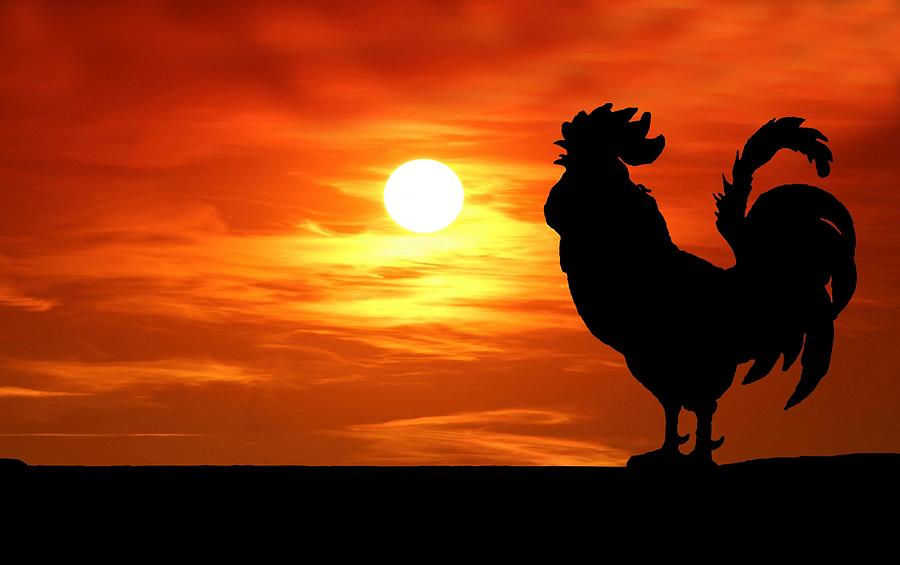A vivid sunrise unfolds in this striking image, with the sky awash in gradients of deep red, orange, and yellow hues. The sun, a prominent bright yellow-white orb, sits near the center, spreading its light outward and giving the scene a mesmerizing glow. The silhouette of the ground is depicted in complete black, creating a stark contrast against the radiant sky. Dominating the right side of the image, a majestic rooster stands tall in silhouette, its defining features—crest, feathers, and talons—clearly outlined in black. The composition places the rooster slightly off-center to the right, leaving the left side of the image unobstructed, further accentuating the expansive, colorful dawn of the new day.